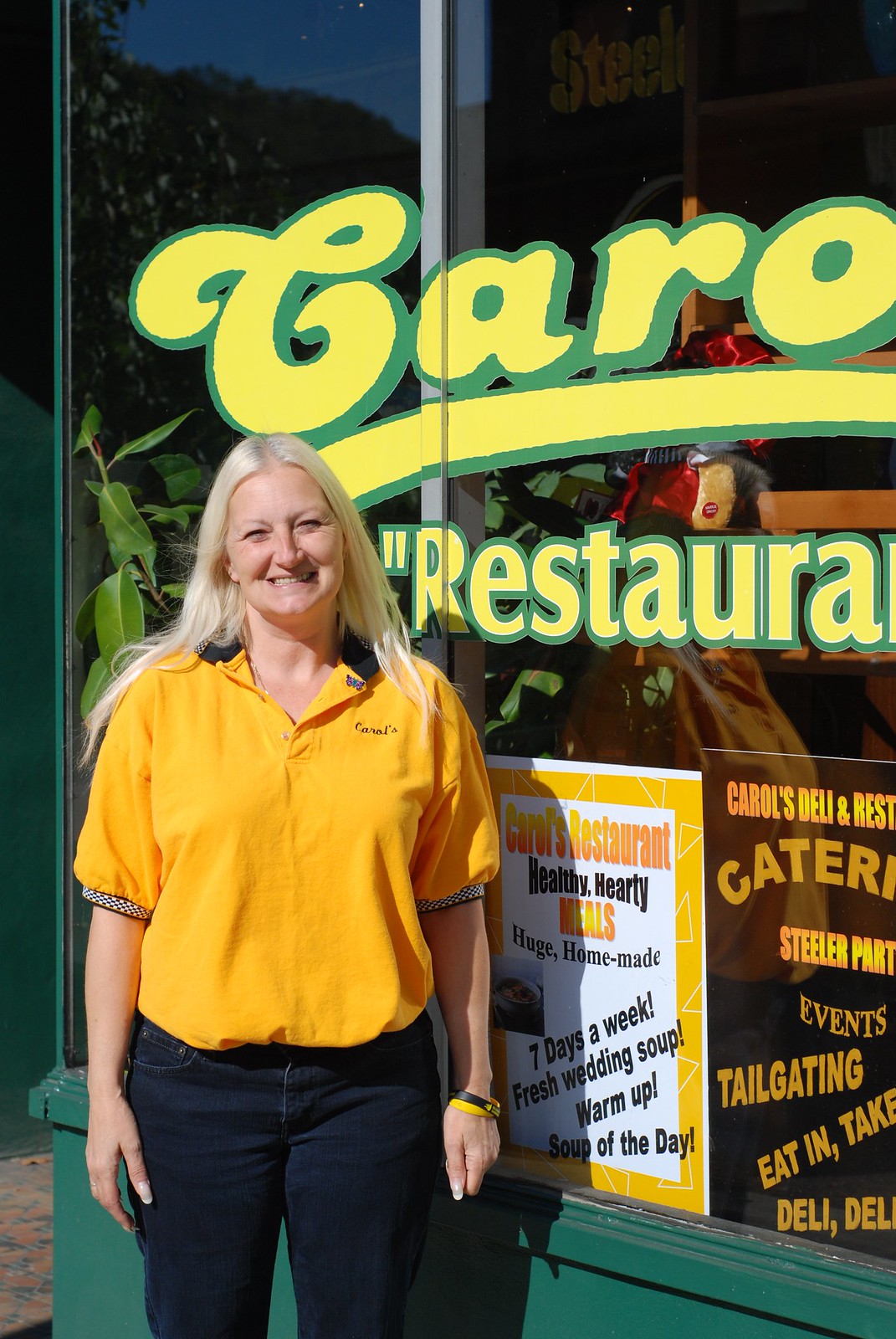In this vibrant and welcoming image, a middle-aged woman with long blonde hair stands smiling directly at the camera in front of a restaurant named Caro Restaurant. The backdrop is a storefront characterized by large glass windows framed in silver, set into a green-colored wall. The windows are painted with a green border and yellow cursive font that reads "Caro Restaurant." The woman, dressed in a bright yellow polo shirt with a black collar and the word "Caro" emblazoned on her chest, pairs her top with dark jeans and wristbands on both wrists. Her attire complements the cheerful and inviting ambiance of the scene. Inside the windows, there are multiple flyers, some reading "Caro's Restaurant: Healthy, hearty meals, huge homemade, seven days a week, fresh wedding soup, warm up, soup of the day," among other enticing menu details. Additionally, plants can be seen inside, adding a touch of greenery to the overall setting. The scene unfolds outdoors, likely in the middle of the day, capturing the essence of this charming and hospitable dining spot.